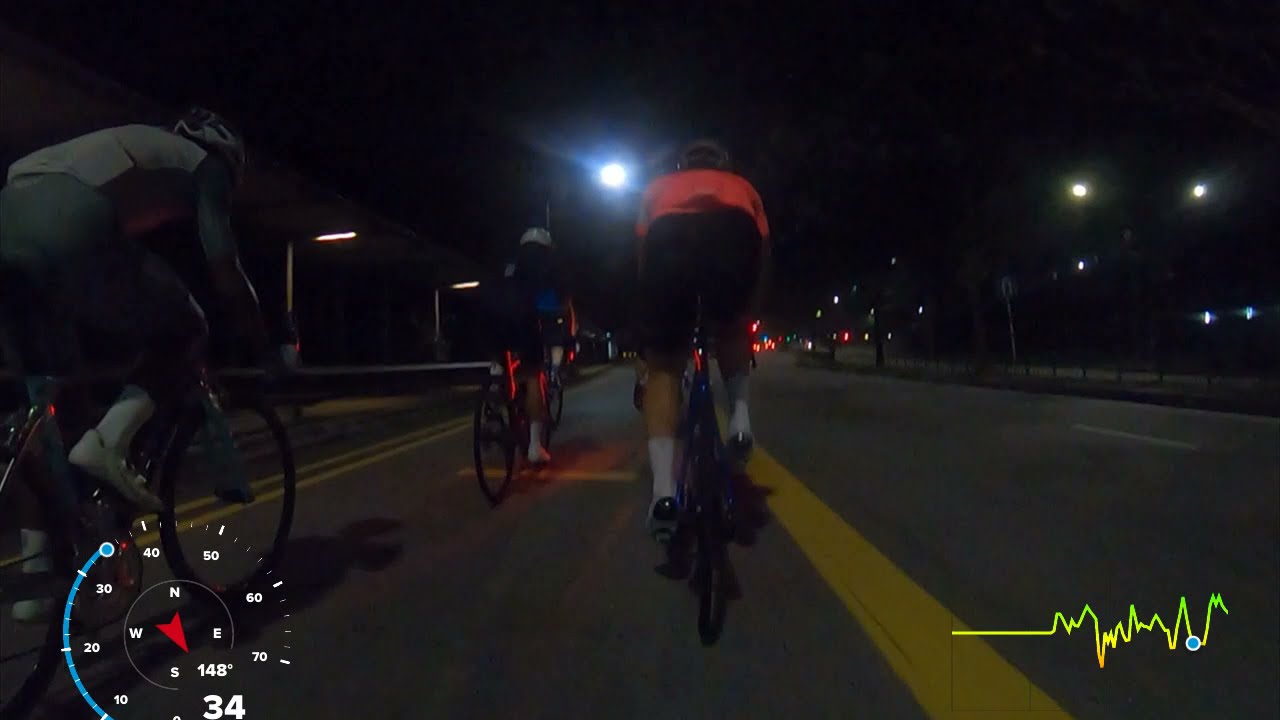This nighttime photo captures three cyclists pedaling along a highway bike lane, their forms illuminated by street lights. The cyclist in the center dons a bright orange shirt, black shorts, and white athletic socks paired with bike shoes. The cyclist to his left, clad in gray shorts and a light gray top, also wears white socks and white bike shoes. Both cyclists sport helmets; the center cyclist has a white helmet, and the left cyclist, a dark one. The bike lane is delineated by a thick yellow line on the right, abutting the main road. In the background, green and red stop-and-go lights are visible. On the lower left corner of the photo, a compass readout indicates we're moving at 34 degrees east-southeast, marked by white text and a red triangle arrow. In the lower right corner, a green line graph against a dark background shows some form of data readout. The photo captures the serene yet industrious atmosphere of bicycling at night, punctuated by the glow of streetlights and traffic signals.